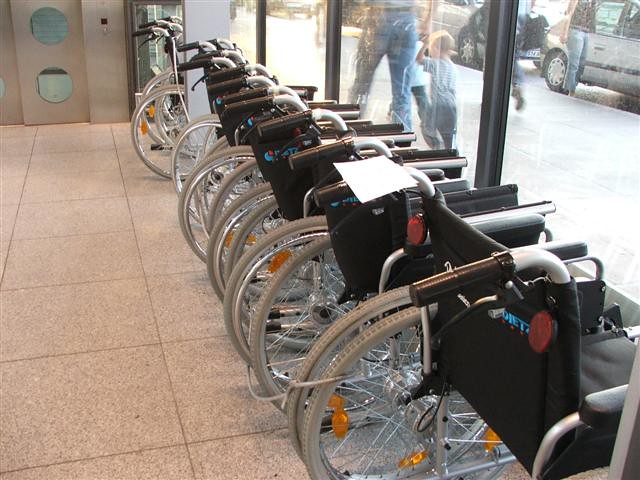In this indoor color photograph, a pristine lineup of brand new wheelchairs draws the viewer’s attention. These wheelchairs, uniformly featuring black seats, silver wheels, and black handles, are aligned along the bottom right-hand portion of the image and extend diagonally towards the top left. Each wheelchair includes reflective elements: red reflectors on the rear and yellow ones within the wheel spokes. A white piece of paper is noticeable on the second wheelchair from the end. The floor beneath them is composed of beige linoleum tiles arranged in a square pattern.

The scene is set within a hospital or a doctor's room, as suggested by the clinical environment. To the right of the wheelchairs, we see a full-length glass wall offering a clear view outside. The glass wall spans from floor to ceiling, interrupted only by a few supporting beams. This expansive window reveals people walking on the sidewalk, including a parent holding the hand of a young child, who appears to be about four years old. There are also cars parked along the street. Further to the left in the upper part of the image, a silver elevator can be discerned, providing additional context to this setting. The photograph captures both the interior precision and the outside activity in a harmonious composition.